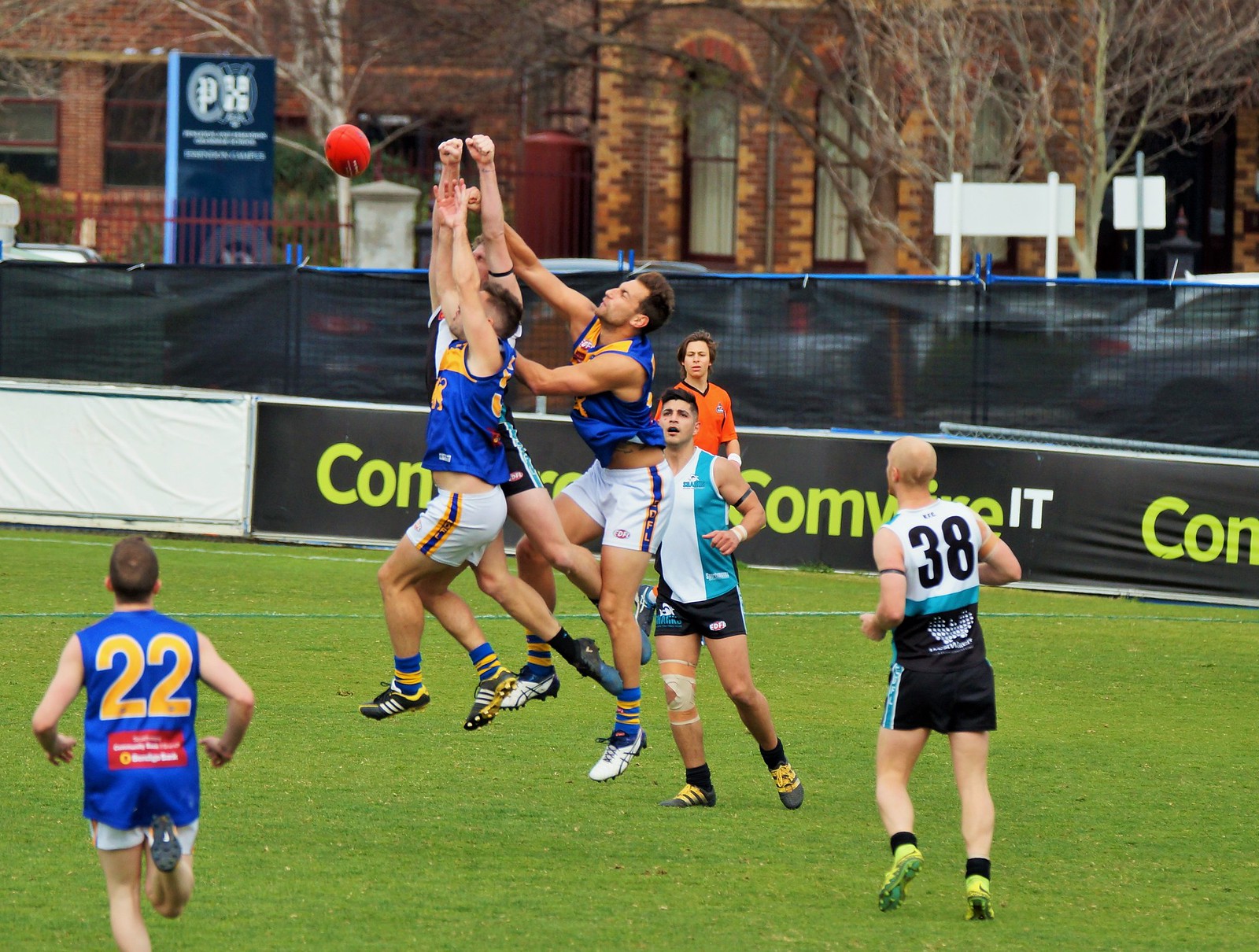In this vivid sports photograph set on a lush green field, we capture a dynamic moment during an intense rugby match in Australia. The focus is on three players from a team in blue sleeveless jerseys adorned with gold numbers, notably including number 22 dressed in white shorts. They leap into the air, attempting to catch a bright red ball. Their opponents, wearing jerseys with white and turquoise vertical stripes and black shorts (featuring number 38), also vie for control of the ball. Adding to the scene, an official in an orange jersey oversees the action. The background features a brick building with a sign in front of it, various fencing, gates, and sponsor banners like the partially obscured "Comvive IT" along the edge of the pitch. The setting is outdoors, further characterized by distant cars, more signage, and a prominent black banner with light green and white lettering.